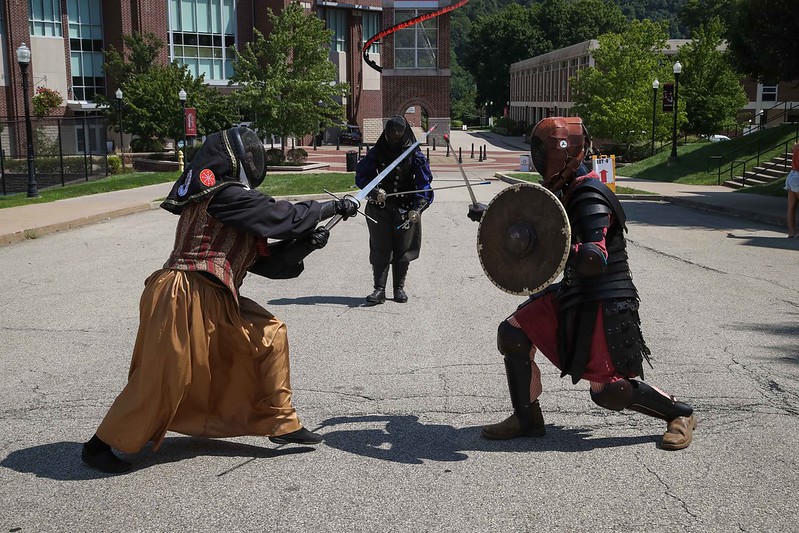In the middle of a courtyard set against the backdrop of university-like buildings surrounded by green trees and sidewalks, a lively medieval sword fight unfolds. The scene, captured in a realistic, horizontally oriented photograph, depicts two figures clad in medieval-style costumes engaging in combat. They both wear protective fencing helmets and light armor to prevent injury. The fighter on the left wears a gold skirt, black shoes, and a red and gold striped vest over a black shirt. Their face is shielded by a black mask with a hard front cover as they brandish a sword. Opposite them, the fighter on the right is dressed in red and black apparel that ends at the knees, with knee-high socks, knee pads, and brown shoes. A red mask covers their face, and in their left hand, they hold a round shield, while their right hand wields a sword. 

Behind the dueling pair, another individual stands observing the fight attentively. This person is also in a dark costume with black boots and a black covering, seemingly playing the role of a referee or judge. The scene is set in the middle of the day, adding an element of vibrancy to the courtyard, which features grass and sidewalks, with a stairway ascending to the right in the backdrop. The image captures a moment of spirited practice or playful combat, blending historical attire and modern surroundings.